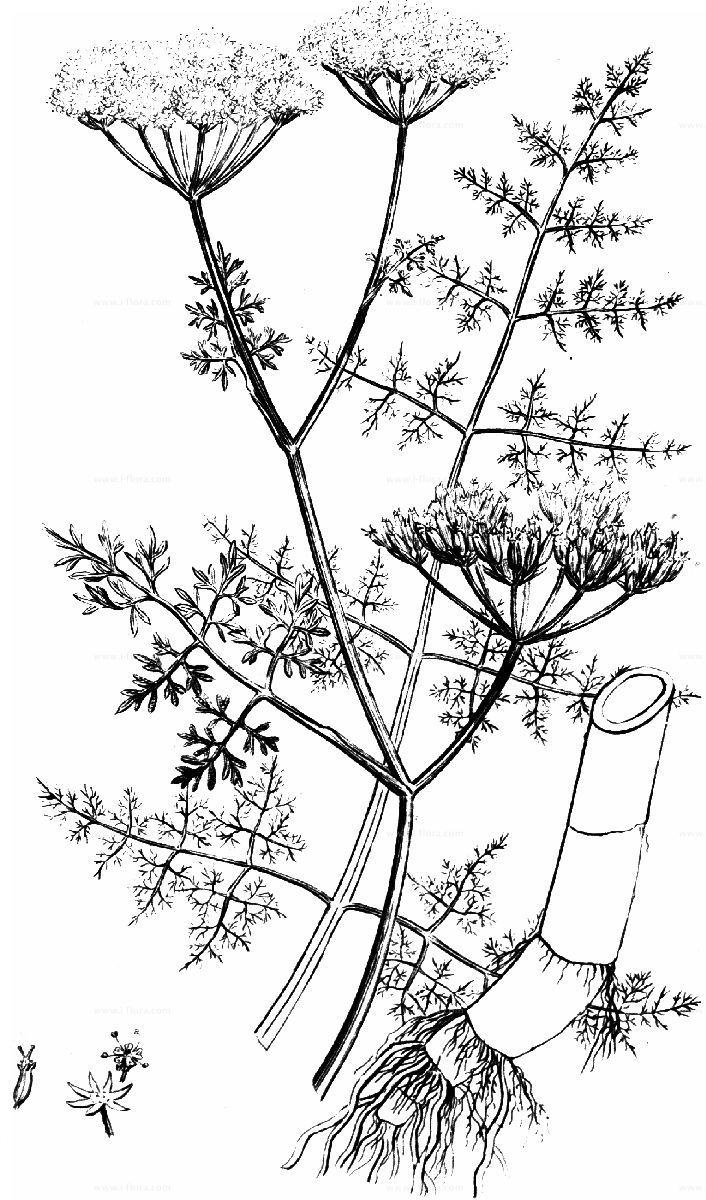This is a detailed black and white scientific drawing, featuring a variety of plants, reminiscent of common wildflowers or weeds. The drawing heavily relies on solid black line work against a stark white background. Predominantly, the image showcases two main plants. 

The first plant in the foreground has a long, slender stem that branches into several clusters of flowers, reminiscent of dandelions. Each cluster contains about eight to ten light-colored flowers. Alongside this main stem, another stem bears a set of fan-shaped leaves that resemble ferns. At the base of the plant, a distinct, tuber-like root system is visible. This segmented, tube-shaped root appears hollow and from each segment, smaller roots sprout out.

To the right, a second plant is depicted with a tall, straight stem that culminates in what appears to be a thin, fern-like structure. This plant emphasizes a vertical growth pattern and in the background, several leafy stems are drawn, creating a sense of depth. 

Additionally, there are smaller renderings of plants on the lower left portion of the drawing. One of these plants features a black stem with a star-shaped top, another resembles a dandelion, and a third has a shape that intriguingly looks like a chili pepper.

Overall, the image captures the intricate details and varying structures of these plants, from their root systems to their flowering tops, providing a rich depiction of botanical life.